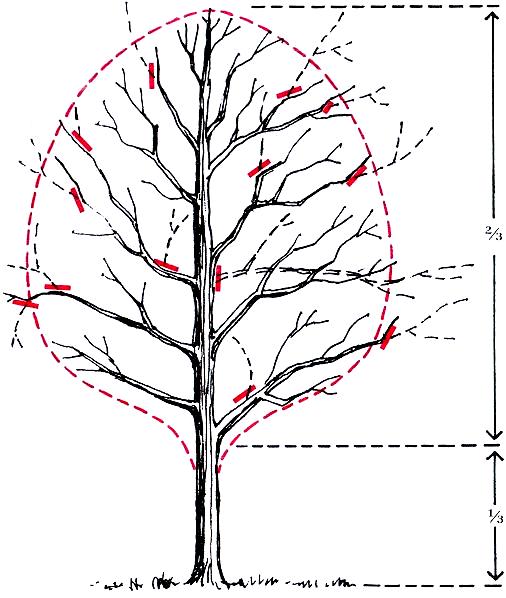The illustration features a meticulously drawn, barren tree situated in the center of the image. The tree's branches, devoid of leaves, are accentuated by dashed red lines that outline the shape of the tree. Scattered across the branches are several small, red, skinny rectangles, implying a specific focus on those areas. To the right of the tree, there are two vertical black lines, each labeled with measurements. The top line, which is longer, is marked "2/3," while the shorter bottom line is labeled "1/3." These lines include arrows and appear to correspond to different sections of the tree. The overall composition hints at an instructional or illustrative purpose, possibly related to teaching a drawing technique or serving as a guide for pruning. The style of the illustration, coupled with its comic-book-like details, suggests it might be designed for educational or artistic contexts.